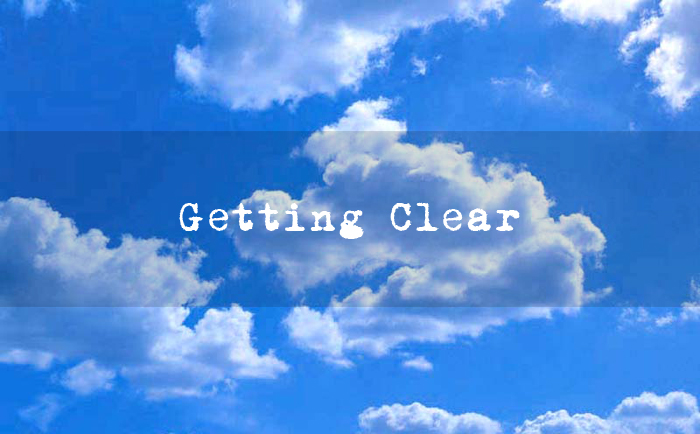This full-color outdoor photograph captures a partially cloudy sky featuring a rich, deep blue gradient that intensifies towards the center. The composition primarily consists of scattered cumulus clouds that add dimension through varying shades of light and shadow. A prominent, semi-transparent horizontal band stretches across the image, occupying approximately one-third of the frame. This band subtly darkens the area behind it and bears the words "Getting Clear" in a vintage typewriter font. The typewriter-like text sits centrally within the band and is deliberately styled to appear slightly blurry, enhancing its nostalgic feel. The rectangular shape of the image is almost square, emphasizing the expansive and vivid atmosphere of the sky. The design elements, specifically the deepened central blue and the overlaying text, appear intentionally digital, creating a striking visual effect.